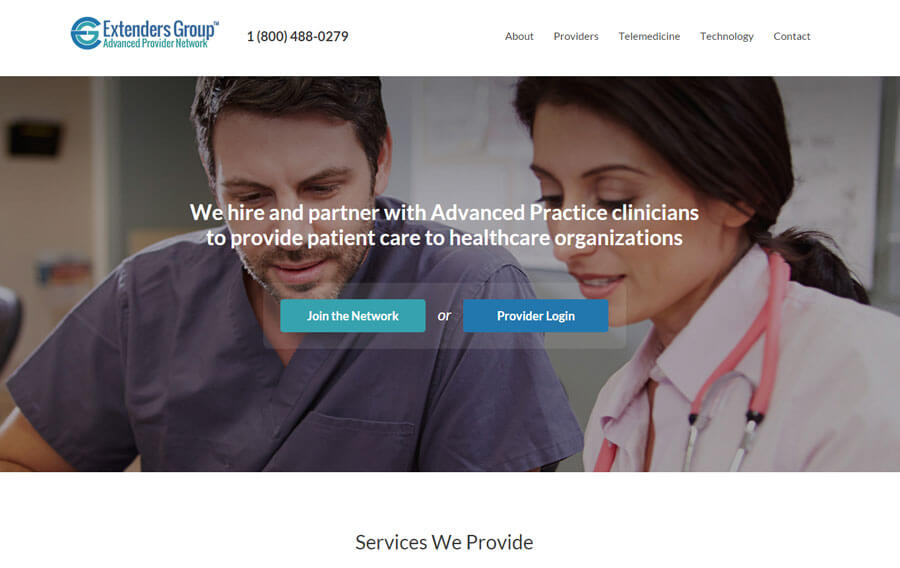In this image, we see a detailed layout of a website page. At the top left corner, the heading "Extenders Group" is displayed prominently. Just below this heading, the text "Advanced Provider Network" is shown in a light blue color. Adjacent to this text, on the right side, is the contact number "1-800-488-0279."

On the right side of the top section, five categories are listed in gray: About, Providers, Telemedicine, Technology, and Contact, all set against a clean white background.

Below this top section, there is a split-screen image featuring two healthcare professionals. On the left side, there is a male doctor wearing gray scrubs, sporting short black hair and facial hair. Only the upper torso, face, and hair of this doctor are visible. On the right side of the screen, a female nurse is depicted wearing a light pink collared shirt with a pink stethoscope draped around her neck. Her black hair is tied back. Both the doctor and the nurse are looking downward in the image.

Centrally placed text reads, "We Hire and Partner with Advanced Practice Clinicians to Provide Patient Care to Healthcare Organizations" in white, superimposed over the images of the professionals.

At the bottom of the image are two clickable options. On the left, a turquoise button with white text reads, "Join the Network." On the right, a blue button with white text says, "Provider Login." 

Finally, at the very bottom of the page, the caption "Services We Provide" is written in gray text. The entire layout is organized neatly, creating a professional and informative visual.